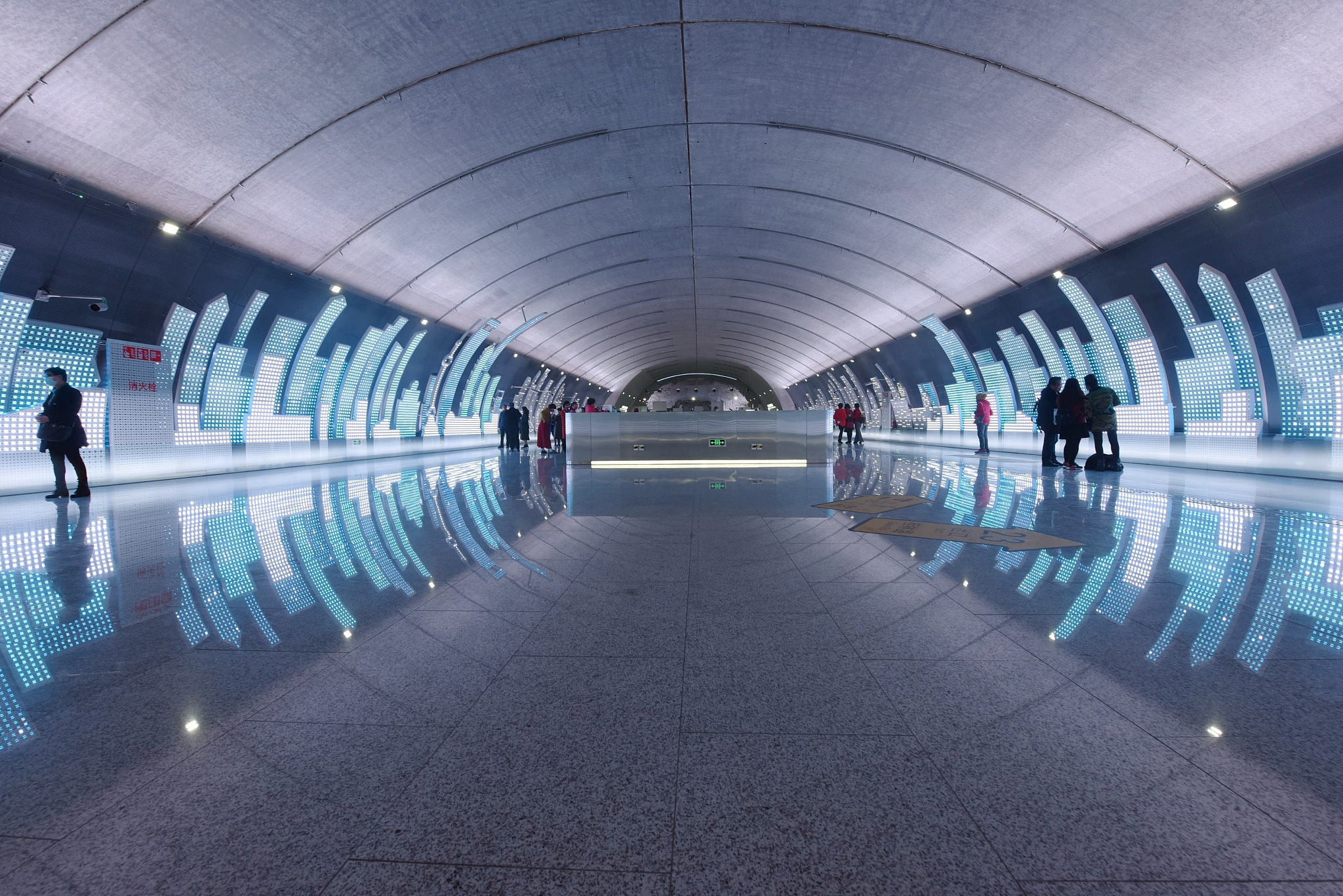The image depicts a photograph of a spacious, high-tech tunnel, possibly in a Chinese metro or airport terminal. The tunnel features a semi-elliptical, domed ceiling tiled in a concrete-like material. The floor consists of gray, rectangular tiles with black grain, separated by thin, dark lines, and is extraordinarily reflective, mirroring the vivid, illuminated surroundings. On either side of the tunnel, an artistic cityscape created from numerous bright white LED lights forms a detailed skyline against a blue background. This cityscape is composed of building shapes that enhance the immersive experience, drawing the attention of the numerous onlookers gathered along the sides. The vibrant display, predominated by blues and whites, casts a colorful glow throughout the corridor, accentuating its modern, futuristic ambiance. The amalgamation of the reflective floor, the curved ceiling, and the intricate illumination gives the tunnel a striking resemblance to a subway or airport terminal, enveloping visitors in a mesmerizing urban spectacle.